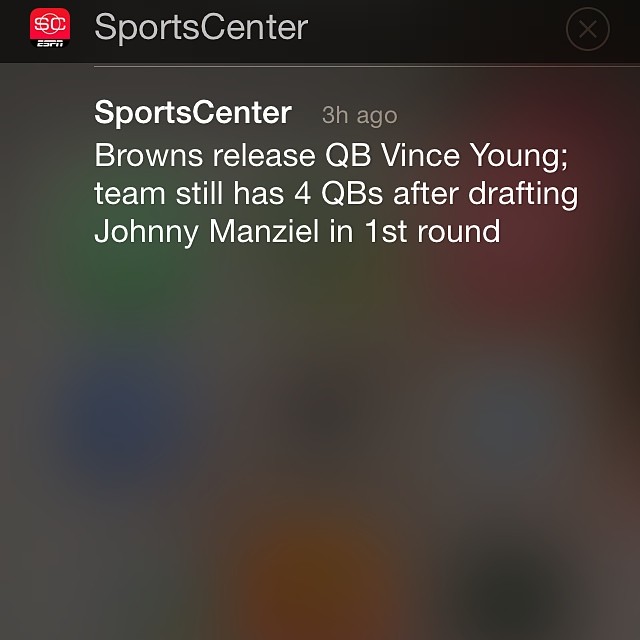The image is a detailed screenshot, likely taken from a mobile device or tablet, displaying a notification from ESPN's Sports Center. The top of the screen features the SC logo—the letters "SC" within a circle with a red background, and "ESPN" underneath in smaller black letters. Adjacent to the logo, the words "Sports Center" are written in white on a black bar, followed by "three hours ago" in gray lettering. The main notification text below, set against a dark gray background, reads: "Browns release quarterback Vince Young. Team still has four quarterbacks after drafting Johnny Manziel in the first round" in white lettering. The image coloration includes black, red, white, gray, orange, green, blue, and light blue. The positioning of the screenshot dominates the entire image frame, and there are faint, indiscernible shapes in the background. The overall presentation is clear, showing text prominently on distinct colored backgrounds, typical of an ESPN notification update.